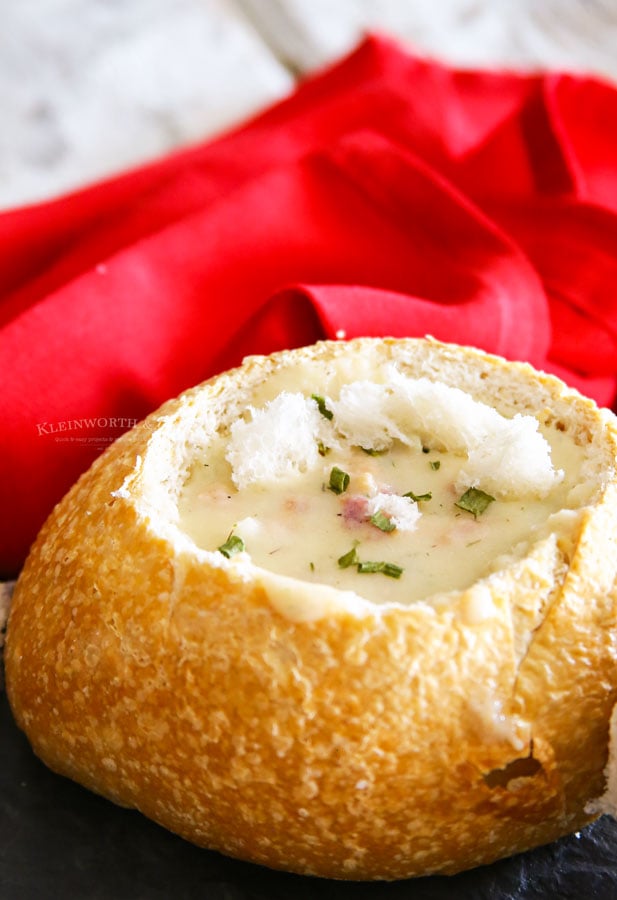A warm, golden-brown bread bowl sits prominently on a dark surface, its outer crust beautifully flaky with small bubble marks indicative of oven baking. Inside, the bowl is hollowed out to reveal its fluffy white bread interior, now filled with a creamy bisque soup. The soup appears beige with hints of pink, likely from chunks of meat, and is garnished with green onion pieces and what might be finely chopped chives. Floating on the surface are small pieces of bread, probably scooped from the bowl itself. Behind the bread bowl, a bright red cloth napkin is crumpled, adding a splash of color, while further back, a blurry white surface suggests a tablecloth. The napkin seems to bear some indistinct gray text, possibly "Keenworth" or "Klein's Wurst." The overall composition captures a delicious and hearty meal setup in a cozy restaurant environment.